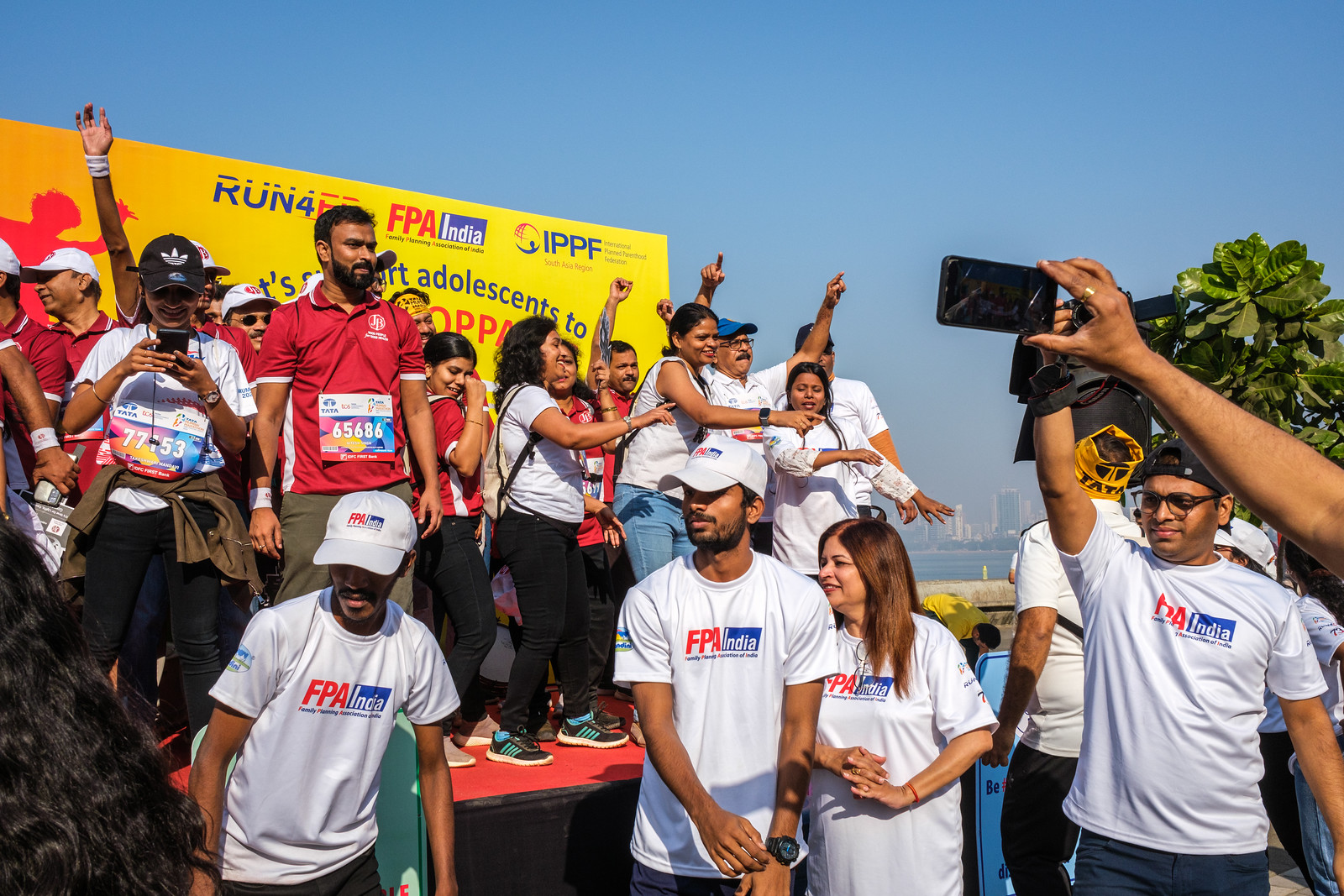This vibrant color photograph showcases an energetic outdoor event in India, primarily featuring a large group of people clad in uniform white t-shirts and caps emblazoned with "FPA India." In the foreground, attendees are standing on the ground, some with phones raised, capturing the moment. Elevated on a platform above them is another group, distinguishable by their red shirts, each adorned with pinned identification numbers, reminiscent of marathon participants. The most prominent figure on this platform is a bearded man with black hair, proudly wearing the number 65686. Behind this platform, a yellow banner reads "Run for Adolescents," flanked by sponsorship logos including FPA India. A scattering of palm trees and a foggy skyline are visible in the distant background, hinting at the proximity of a river. The overall composition suggests that this is a community event centered around a road race, with spectators and participants alike united in their enthusiasm.